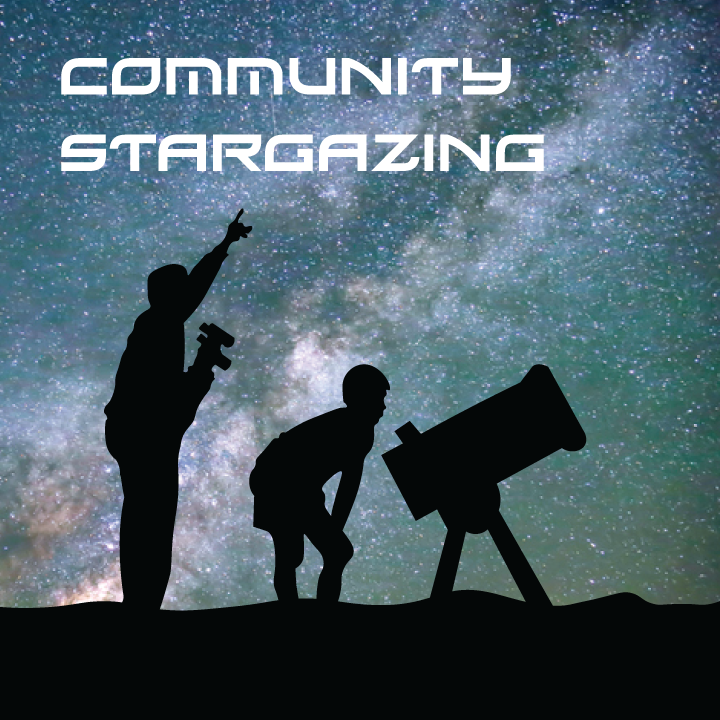The poster features a striking Milky Way backdrop that occupies three-quarters of the image, transitioning into a wavy, black silhouette of a hill at the bottom. At the top, in bold, white, science-fiction-inspired font aligned to the left, the text reads "Community Stargazing." This text evokes a 1950s retro style. In the foreground, silhouetted against the starry night, is a scene of two figures engaged in stargazing. A young boy is leaning forward with his hands on his knees, peering into a large, stocky telescope mounted on a tripod. Behind him stands a man, holding binoculars in his right hand and pointing upwards, possibly illustrating a constellation for the boy. The figures are rendered as black silhouettes, emphasizing their focus on the celestial wonders above. The overall impression is a blend of photographic and hand-drawn elements, highlighting a communal activity centered around exploring the night sky.